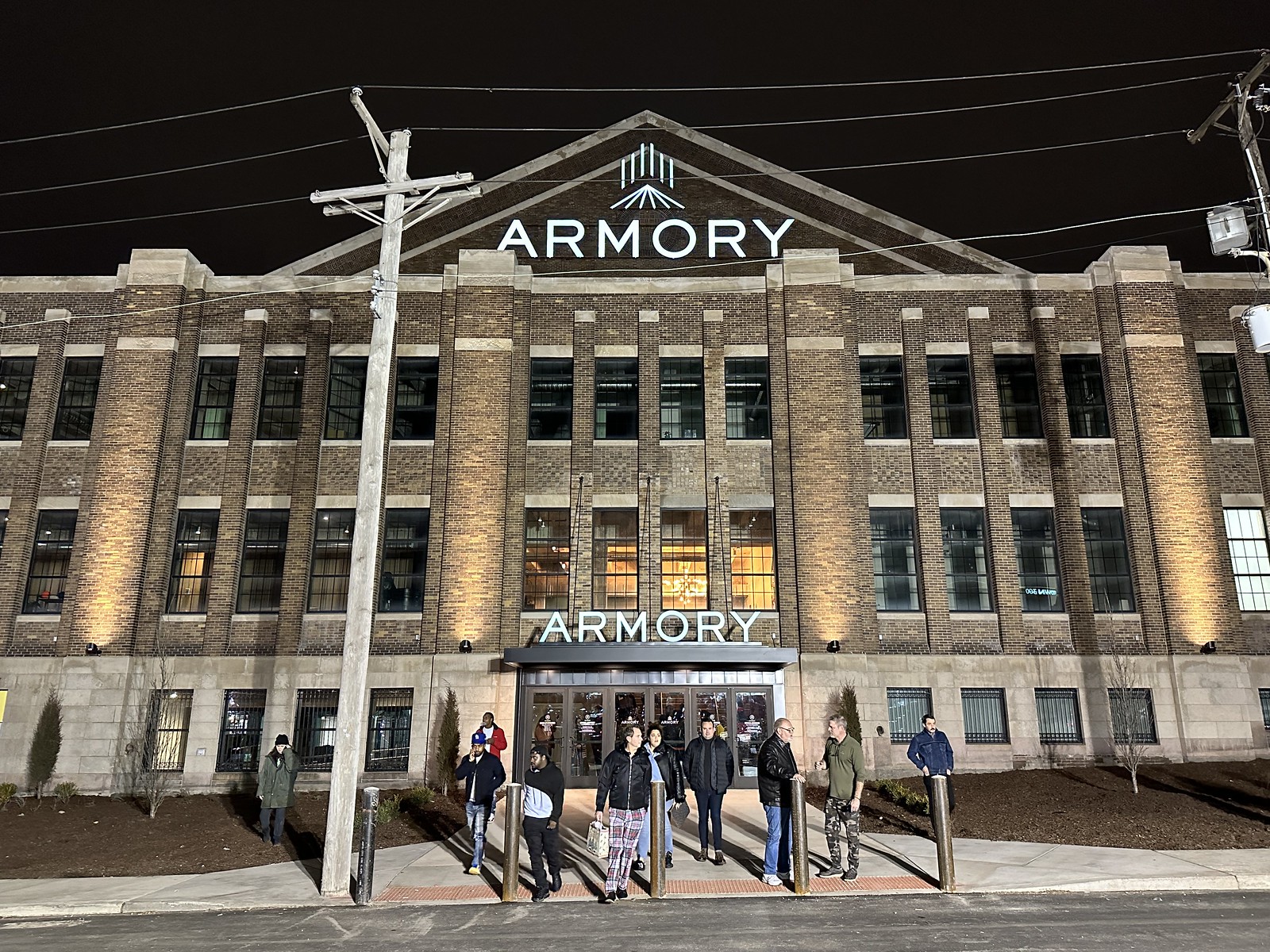This nighttime photograph captures an impressive armory building made of brown brick and stone, rising three stories high. The structure boasts a pronounced triangular roof with the word "Armory" prominently displayed in big white letters. Below the roof, grand columns extend down to the second floor, which also features the "Armory" text again in white. The front facade is beautifully illuminated by spotlights, highlighting its robust architectural elements. 

Centered at the front, under a black overhang roof, are three sets of black double doors flanked by windows on either side. The entrance area is bustling with several people clad in fall attire, including long sleeves and light coats. Some individuals are conversing while others appear to be waiting, possibly for a bus. Among them, a man carrying a bag stands out. 

In front of the building, the sidewalk is bordered by five short posts preventing vehicles from crossing into the pedestrian area. There's also a prominent utility pole on the left side with wires extending across the scene, adding to the urban realism. The sidewalk leads up to the street, where small patches of dirt flank either side.